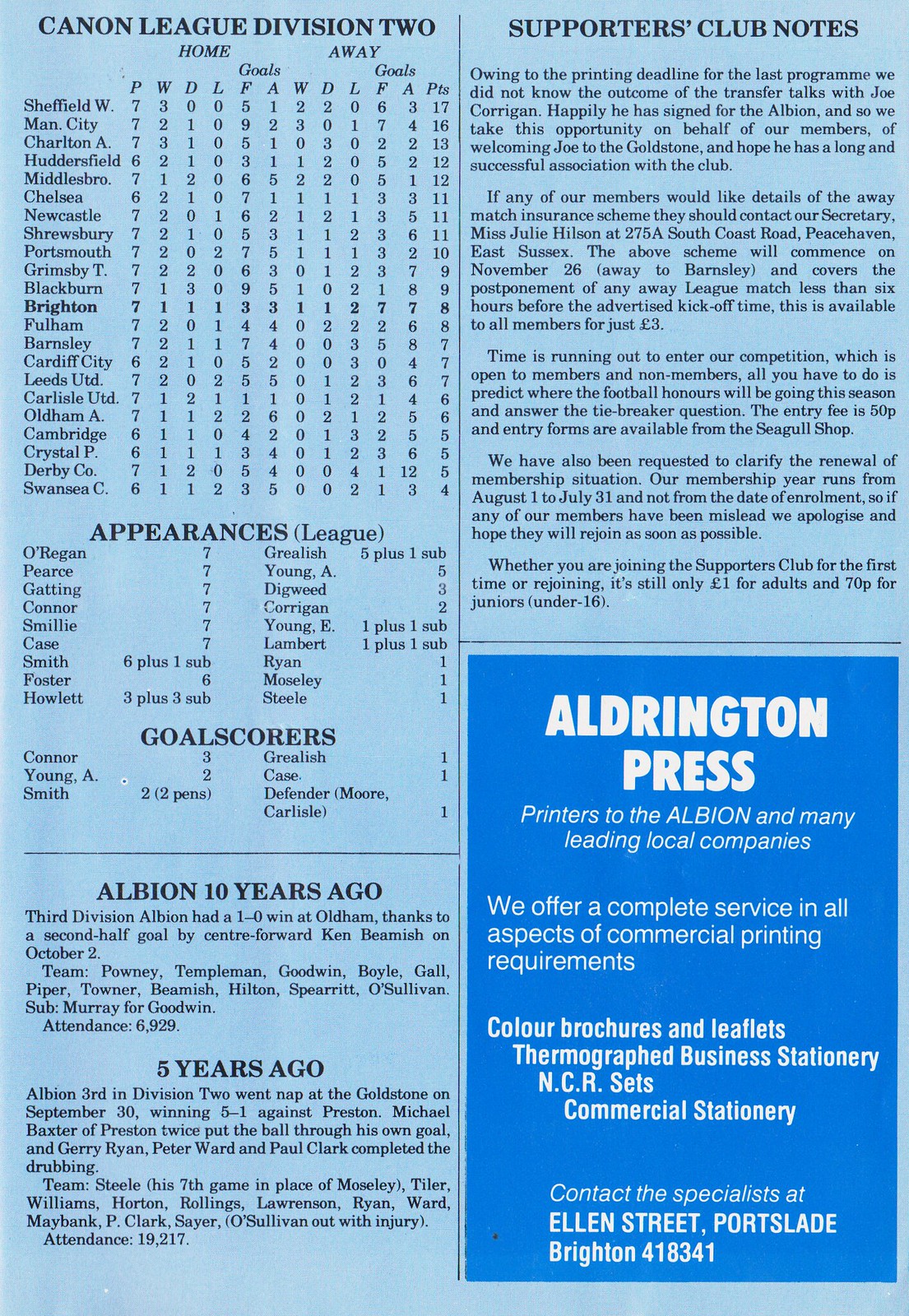The image is a rectangular program, approximately six inches tall and four inches wide, with a periwinkle blue background. It is divided into a left and right section. The left section is further divided into a larger top portion, taking up about two-thirds of the page, and a smaller bottom portion. The right section is divided into two equal halves.

In the top portion of the left section, bold black print reads "Cannon League Division 2," and includes columns labeled Home, Away, and Goals. The names of football clubs such as Sheffield, Manchester City, Charlton, Huddersfield, Middlesbrough, and Chelsea are listed here, along with their respective goal statistics for home and away games. A subsection below this is dedicated to player appearances and goal scores, further detailing individual player statistics and their jersey numbers.

The bottom portion of the left section features historical content, with two distinct paragraphs: one about Albion from 10 years ago, and another about Albion from 5 years ago.

The right section has two parts. The top portion is labeled "Supporters Club Notes," providing information pertinent to the club's supporters. The bottom portion is dark blue with white text, displaying an advertisement for Alderton Press, which reads: "Printers to the Albion and many leading local companies." It elaborates on the services offered by the company, including color brochures, leaflets, and various types of commercial stationery, and provides their contact details at Ellen Street, Port Slade, Brighton, with the phone number 418-341.